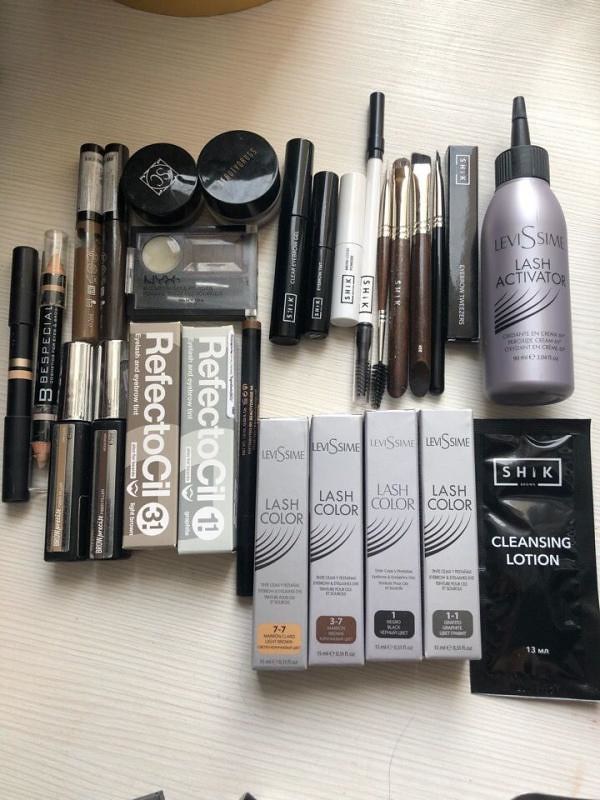The close-up photo captures an assortment of makeup utensils arranged on a white wooden tabletop. Dominating the bottom right of the image is a black package with "Chic" written in a white rectangle, reminiscent of magazine sample packs, labeled "cleansing lotion" in white text. Next to it, four identical boxes labeled "lash color" display shades of blonde, brown, black, and gray. Further left, the image features two ReflectoSol products: ReflectoSol 1 in gray packaging and ReflectoSol 3 in brown packaging. Additionally, a silver plastic bottle with a black tip, labeled "Lash Activator," appears ready for dispensing. Scattered around are various brushes and what seems to be a collection of either eyeshadows, brow pencils, or lip pencils, although their exact identities are indeterminate.